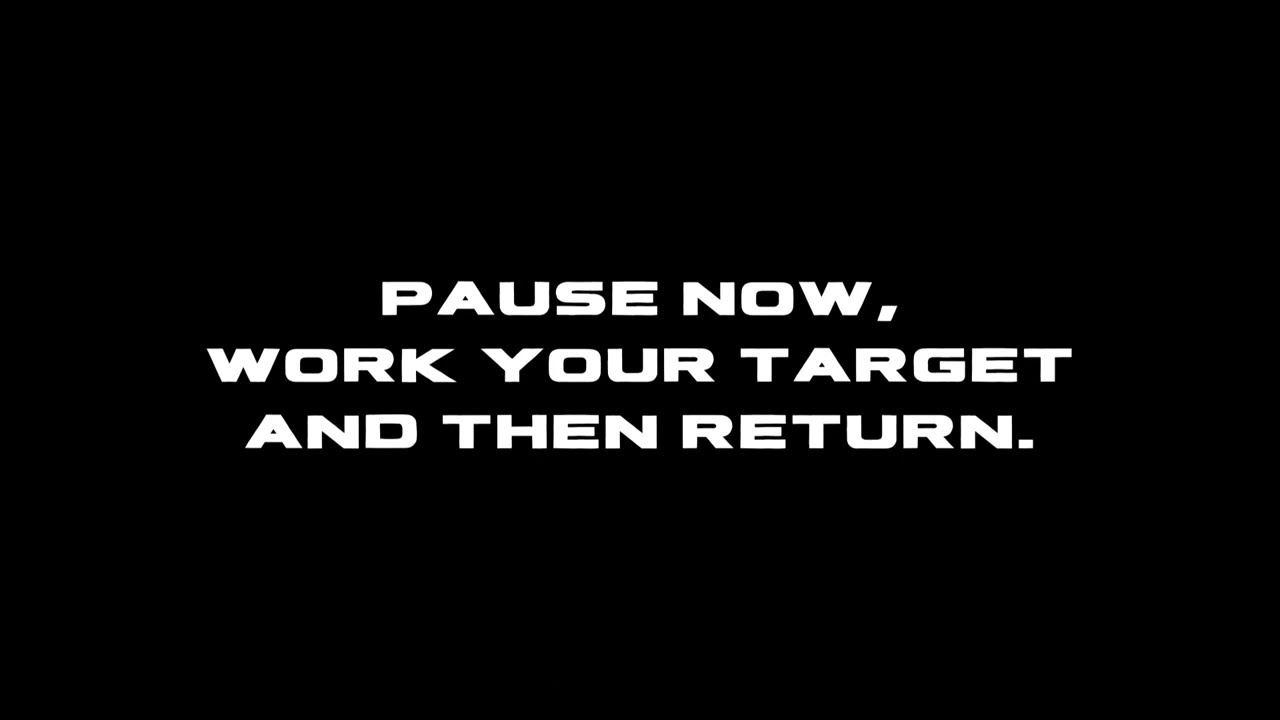This is a simple yet striking image, prominently featuring white, all-caps block letters against a solid black background. The message is presented in three centered lines of horizontally compressed typeface. The first line reads "PAUSE NOW," followed by a comma. The second line, extending further to the left and right than the others, instructs "WORK YOUR TARGET." The final line concludes with "AND THEN RETURN," terminated with a period. The uniformity in the font style and color across the entire image highlights its graphic and instructional nature, possibly resembling a still from an instructional video or a minimalist informational poster.